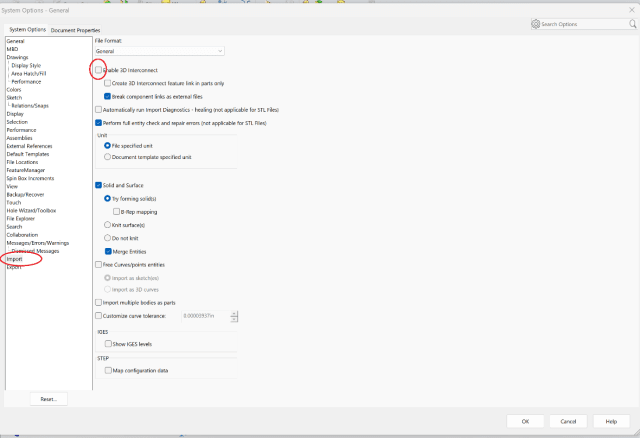This horizontal, left-to-right image depicts a computer screen with a predominantly black background. At the very top, there are some partially visible icons, with notable labels including "System" and "Optos General." A gray 'X' icon is prominently positioned towards the upper right-hand corner, just below a row featuring a settings icon, magnifying glass, and search options.

On the left-hand side, the screen is split into sections with various labels in black font: "General," "Drawings," "Display Style," "Colors," "Sketch," "Display," "Performance," "Assemblies," "External Performance," "Default Templates," "File Locations," "Features Manager," "View," "File Explorer," "Search," "Collaboration," "Messages," "Errors," and "Warnings." Among these, the word "Import" stands out with a red circle around it, while "Export" is located directly below.

To the right, the phrase "File Format is General" is visible, highlighted by a circle around an unchecked box labeled "Enable 2D Interconnect." Below this, several checkboxes display a mix of blue-checked and unchecked statuses.

At the bottom right-hand corner of the screen, there are three buttons labeled "OK," "Cancel," and "Help," providing options for the user to proceed, cancel the operation, or seek assistance.